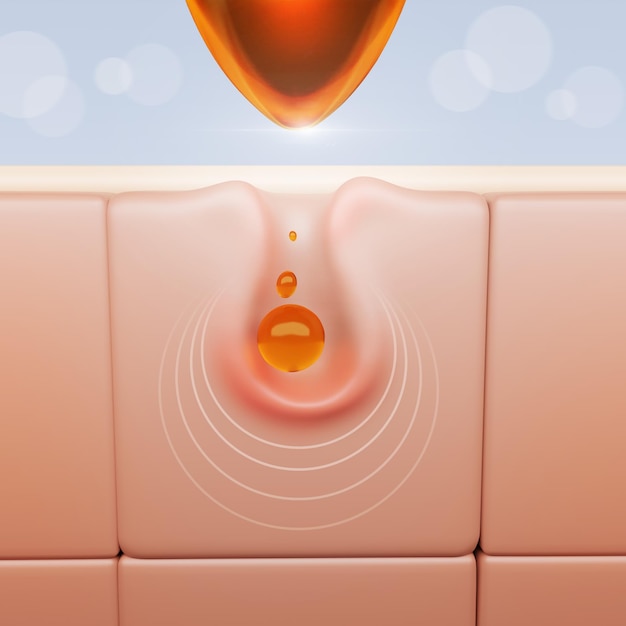The image is an AI-generated or illustrated abstract visual depicting three flexible, pink, spongy square shapes, resembling leather cushions or possibly skin cells. The squares are stacked in two layers, with a noticeable indentation in the center square. Above this indentation hovers an orange, pin-shaped object, which appears to be dripping orange droplets into the indented square. The drops are clearly visible in the indentation, enhancing the sense of depth and interaction. Surrounding the indentation are four white semicircular lines, suggesting movement or pressure. The background is a calming blue with scattered white bubbles or lens flare effects, contributing to the overall abstract and complex nature of the scene.